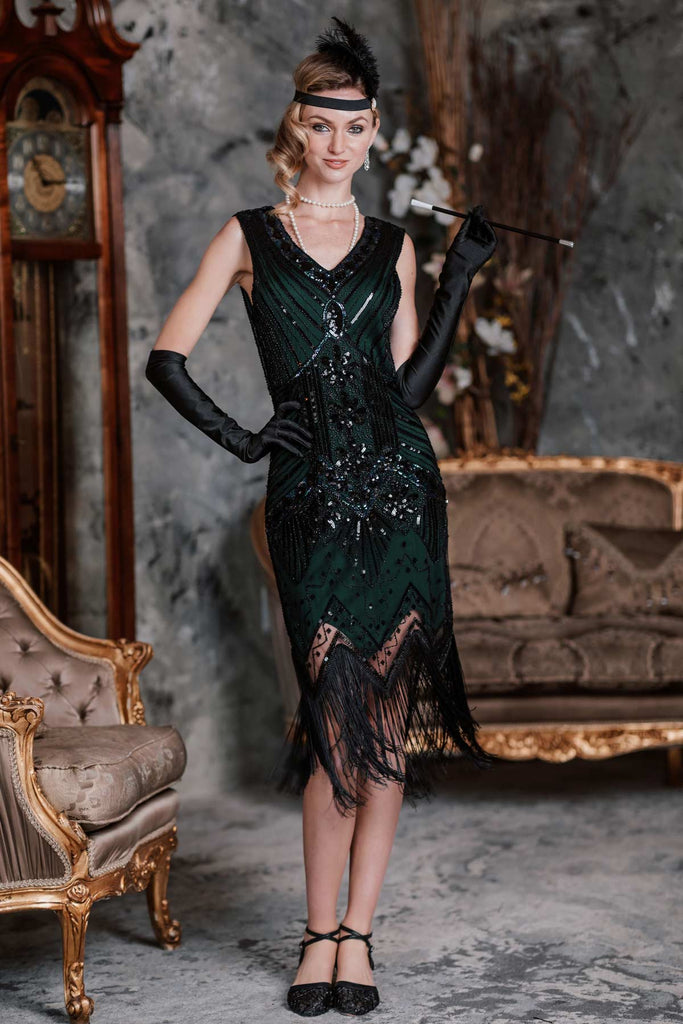In this striking, crisply detailed photograph, a young woman exudes the elegance of the Roaring Twenties. She stands confidently in a room with gray carpet and marble-esque gray walls, posing for the camera as though preparing for a night out. She wears a stunning black sequined flapper dress, adorned with a dark green, black overlay, and black fringe at the bottom. Her sleeveless dress features a V-neckline, perfectly complemented by long black gloves extending past her elbows.

Her accessories further enhance her vintage look: she holds a long cigarette in a black holder, and her forehead is encircled by a black headband with a feather. Her hair is styled up with tendrils cascading down the right side of her face, accentuating her black-lined eyes and delicate white beads around her neck. On her feet, she sports black flat shoes with a crisscross design at the ankle.

The backdrop includes French Regency-style furniture, including a brown couch with gold trim, and a chair to her right. Behind her stands a mahogany grandfather clock, its hands pointing to 10:15, and tall reeds with floral accents add a touch of nature to the scene. The room's harmonious blend of antique and natural elements enhances the authenticity of this meticulously crafted period portrait, perhaps created using AI technology.